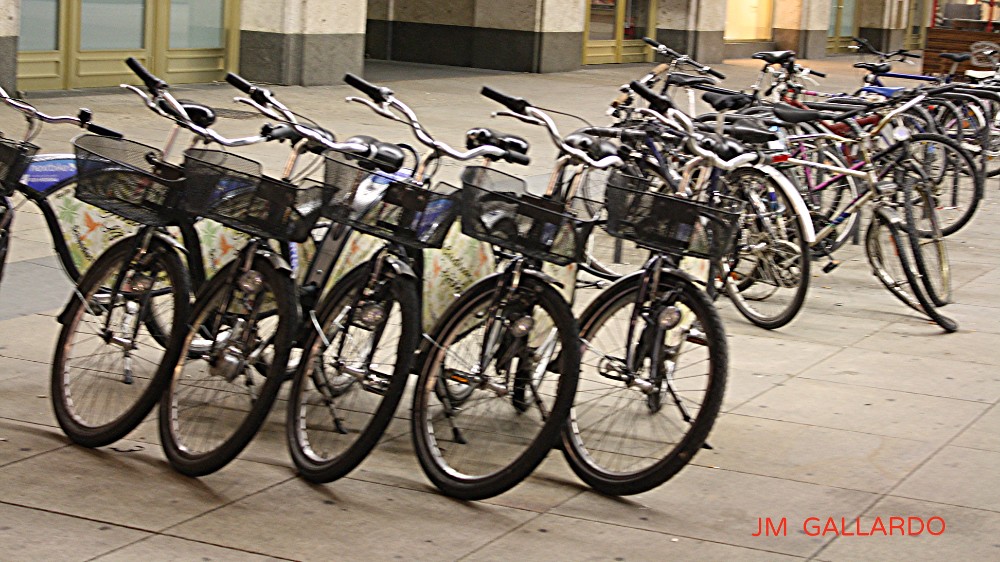This photograph showcases a bustling outdoor walkway with a collection of approximately 25 to 30 bicycles, which are parked in an orderly manner on white, large tiled surfaces. In the forefront, there are six nearly identical bicycles with rectangular baskets, black wheels, and silver and black handlebars, adorned with papers featuring green plant-like symbols and flags with orange and blue accents. Additional bicycles, displaying slight variations in color—mainly black, white, silver, with occasional pink, red, and blue—extend into the background on the right, some of which have bent wheels. Behind the bikes stands an elegant building characterized by its gray stonework on the lower portion and white above, golden doors with large windows, and various entrances visible. At the bottom right corner of the image, the name "J.M. Gallardo" is prominently displayed in red lettering.